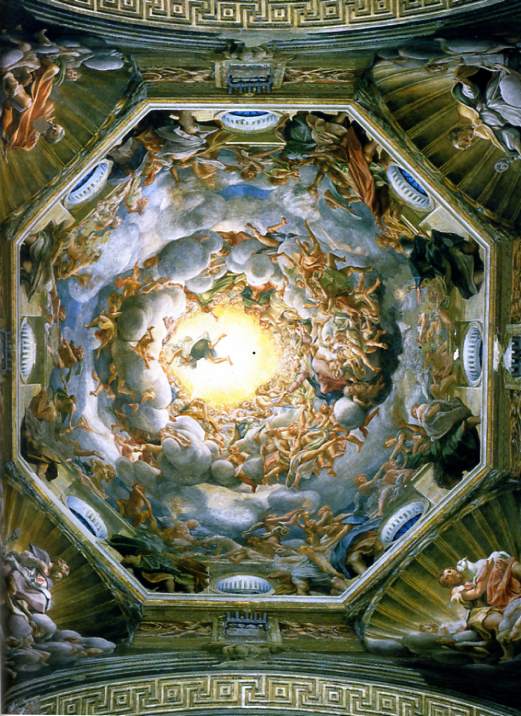This detailed photograph showcases the elaborate ceiling of a domed church, captured from directly below, allowing us to gaze upward into the intricate mural above. Dominating the ceiling is a massive, ornate octagonal mural that evokes a celestial scene. Within this octagon, we see an ethereal representation of heaven, filled with swirling white clouds that spiral towards the center, becoming narrower as they converge into a radiant yellow and white light, symbolizing the heavenly realm. Scattered throughout the spiraling clouds are numerous human figures, depicted in various states; some are fully legged while others are enveloped in flowing fabric, seemingly ascending or struggling against the pull towards the luminous center.

Each of the four corners of the mural features distinct biblical images, adding to the religious profundity of the artwork. The meticulous design of the mural creates an illusion of movement, with people appearing to be swept up towards the heavenly light, akin to the eye of a gentle, divine vortex. Additionally, a white circular opening on each side of the octagon complements the scene, each adorned with a unique cut-out element. The antiquated style of the mural suggests it dates back to the 1500s, giving it a timeless, historic feel.